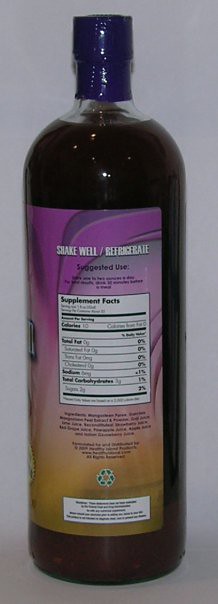The image captures a color photograph in portrait orientation, focusing on a long gray rectangle as the backdrop. In front of this rectangle stands an unopened bottle filled with a dark brown liquid, resembling soy sauce. The clear bottle has a distinctive blue cap, secured with an unbroken plastic seal. The label on the bottle transitions from purple at the top to orange at the bottom and includes various details: "Shake Well / Refrigerate," suggested use instructions, and supplemental facts. The front of the label is turned away, revealing only the general and supplementary information printed on a white section near the bottom of the bottle. This suggests that the bottle contains some type of dietary supplement.